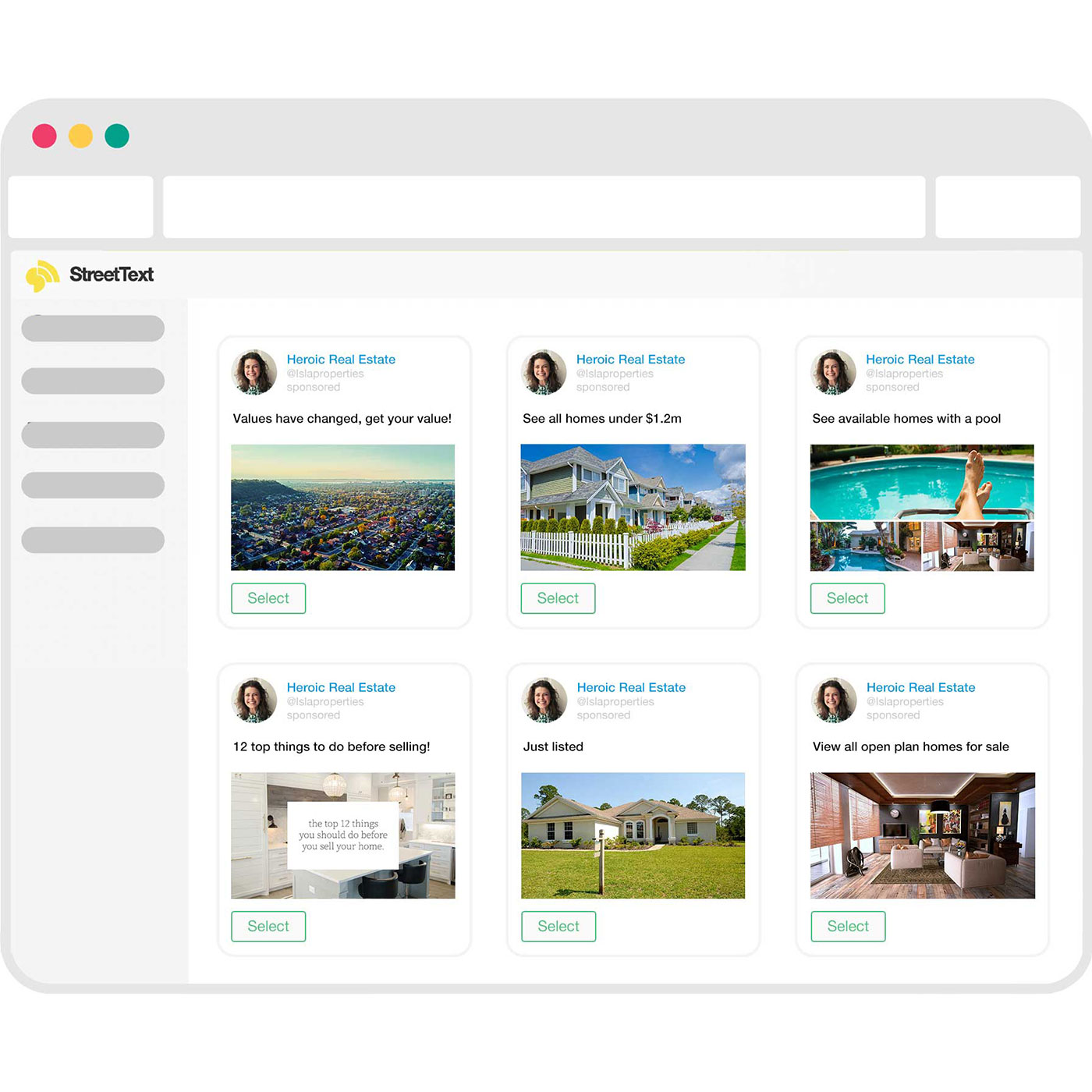This is a detailed mock-up of an application called "Street Text," presented in a browser interface with a gray background. At the top left of the browser, there are three colored dots: red, yellow, and green, mimicking a control panel for closing, minimizing, and maximizing the window. Directly beneath these dots, there are blank white spaces designated for search box logos, following which lies the search input area.

The webpage is divided into two main sections. On the left side, there is a vertical gray panel filled with blank gray spaces, which are placeholders symbolizing different categories. At the very top of this panel is the title "Street Text."

The right side of the mock-up represents the main body of the webpage. This section has six thumbnails displayed in a format akin to tweets, all originating from the same real estate agent. Each thumbnail includes a profile picture at the top left corner. To the right of the picture, the agent's name and additional information are displayed. Just below this, there is a short message, the first of which reads, "Values here have changed, get your value." Each message is accompanied by a thumbnail image showing an aerial view of a city. To the right of each message and image, there is a selectable button labeled "Select." All six thumbnails follow this consistent format: the agent's name and profile picture at the top, an informational message with a thumbnail image below, and the "Select" button to the right.